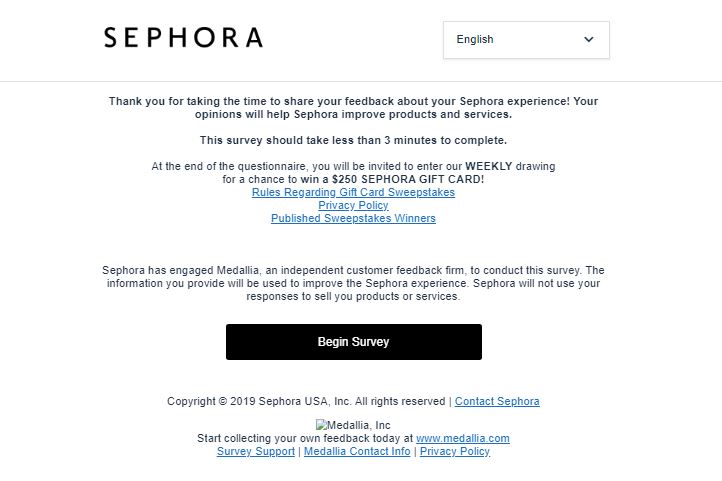The image is a screenshot of a Sephora webpage designed to gather customer feedback through a survey. At the upper left-hand corner, the word "SEPHORA" is prominently displayed in large, bold black uppercase letters. To the right of the Sephora logo is a language selection bar labelled "ENGLISH," allowing users to choose their preferred language for the page content.

Centered below this header, there's a message thanking users for taking the time to share their feedback about their Sephora experience. The text emphasizes that their opinions are valuable in helping Sephora improve its products and services. The message continues to inform participants that the survey will take less than 3 minutes to complete.

Further down, there's an additional note mentioning that at the end of the questionnaire, respondents will have the opportunity to enter a weekly drawing for a chance to win a $250 Sephora gift card.

Beneath this, there are three hyperlinks stacked vertically: the first one gives information on the "rules regarding gift cards sweepstakes," the second one links to the "privacy policy," and the third one allows users to "publish sweepstakes winners."

At the bottom of the page, there is a prominent "Begin Survey" button, inviting users to start the feedback process.